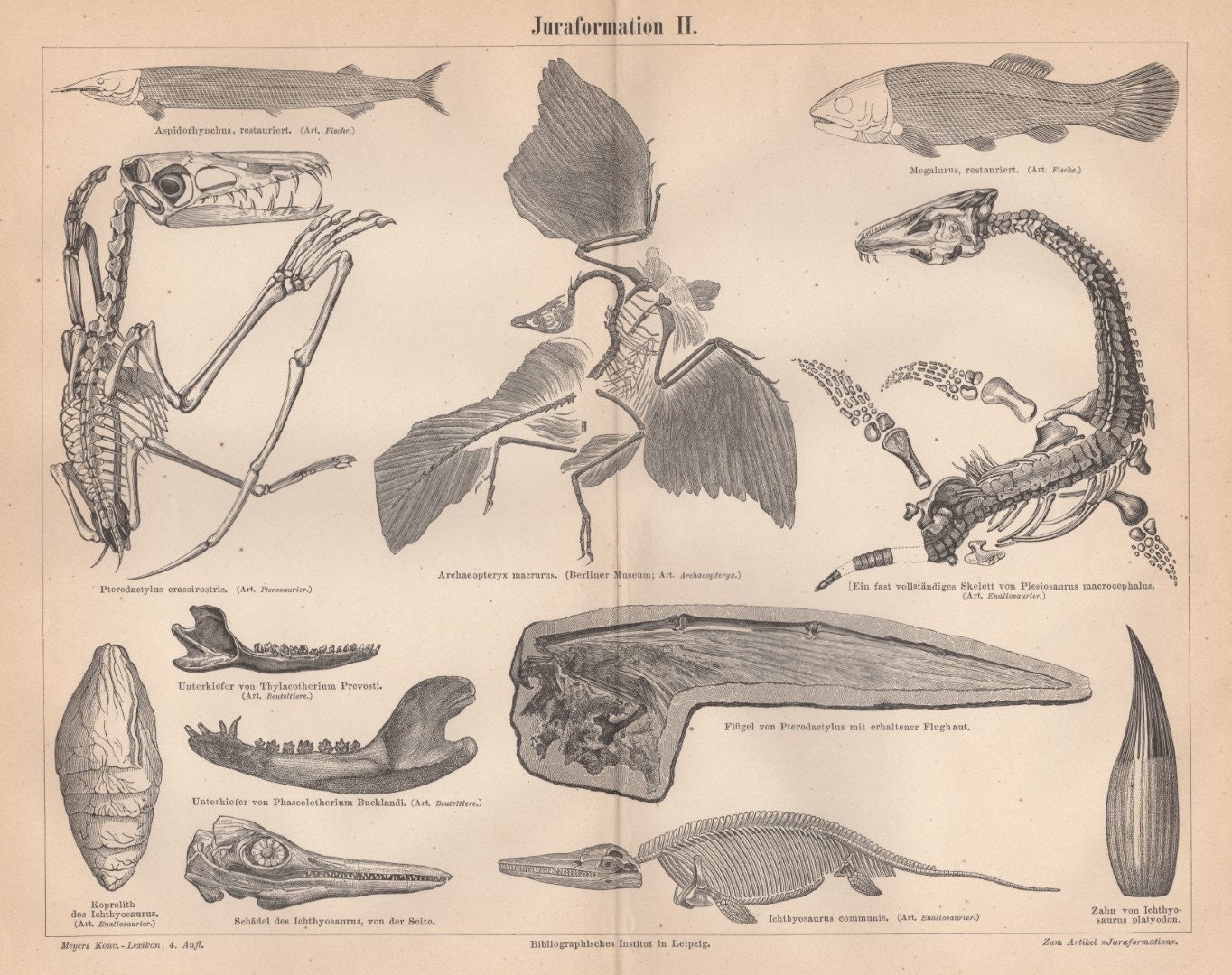This image is a detailed antique fossil print, appearing to be a page from an old book, evidenced by the prominent crease down the center. The page, tinged with a brown, aged hue, features finely drawn depictions of various prehistoric fossils and bones in dark black or gray ink. Dominating the center is an Archaeopteryx, a bird-like dinosaur with feathers, displayed alongside its skeleton. Below this is the fossil of an Ichthyosaurus, a fish-like reptilian skeleton. The page also showcases an array of other prehistoric creatures, including a long, slender fish, a smaller fish, and what appears to be a pterodactyl or similar bat-like bird dinosaur. Among the illustrated fossils are jawbones, seashells, cocoons, and a striking giant claw. Although some figures are indistinguishable, the detailed representations serve as an identification guide to various ancient species. The image includes some text, albeit difficult to read, with a caption at the top mentioning "Jura formation number two." This print exemplifies a meticulous and educative portrayal of ancient fossils, valuable for understanding and identifying prehistoric remains.